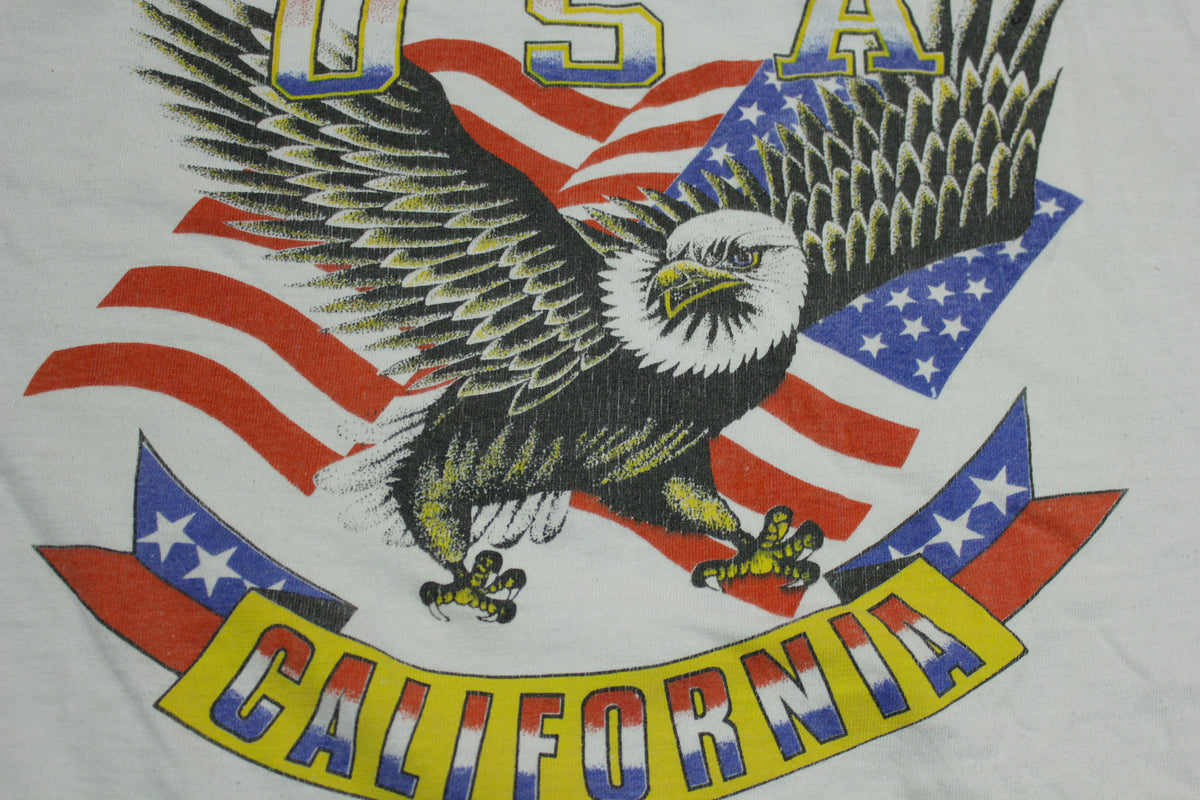The image depicts a dynamic American Eagle artwork overlaid on an American flag, with a white background. At the top, it prominently says "USA" in white lettering that fades into blue at the bottom of each letter. Below, a yellow banner arched upward displays the word "California" in bold red, white, and blue letters. The eagle, with its white head and neck, is flying towards the right while looking left. Its outstretched wings and extended talons give it a poised, predatory stance as if about to grasp something. The eagle's sharp talons prominently extend over the yellow banner. Surrounding the eagle are three stars on either side of its wings. The background includes blue fields with white stars at the top and red stripes at the bottom, completing the American flag imagery behind the eagle.